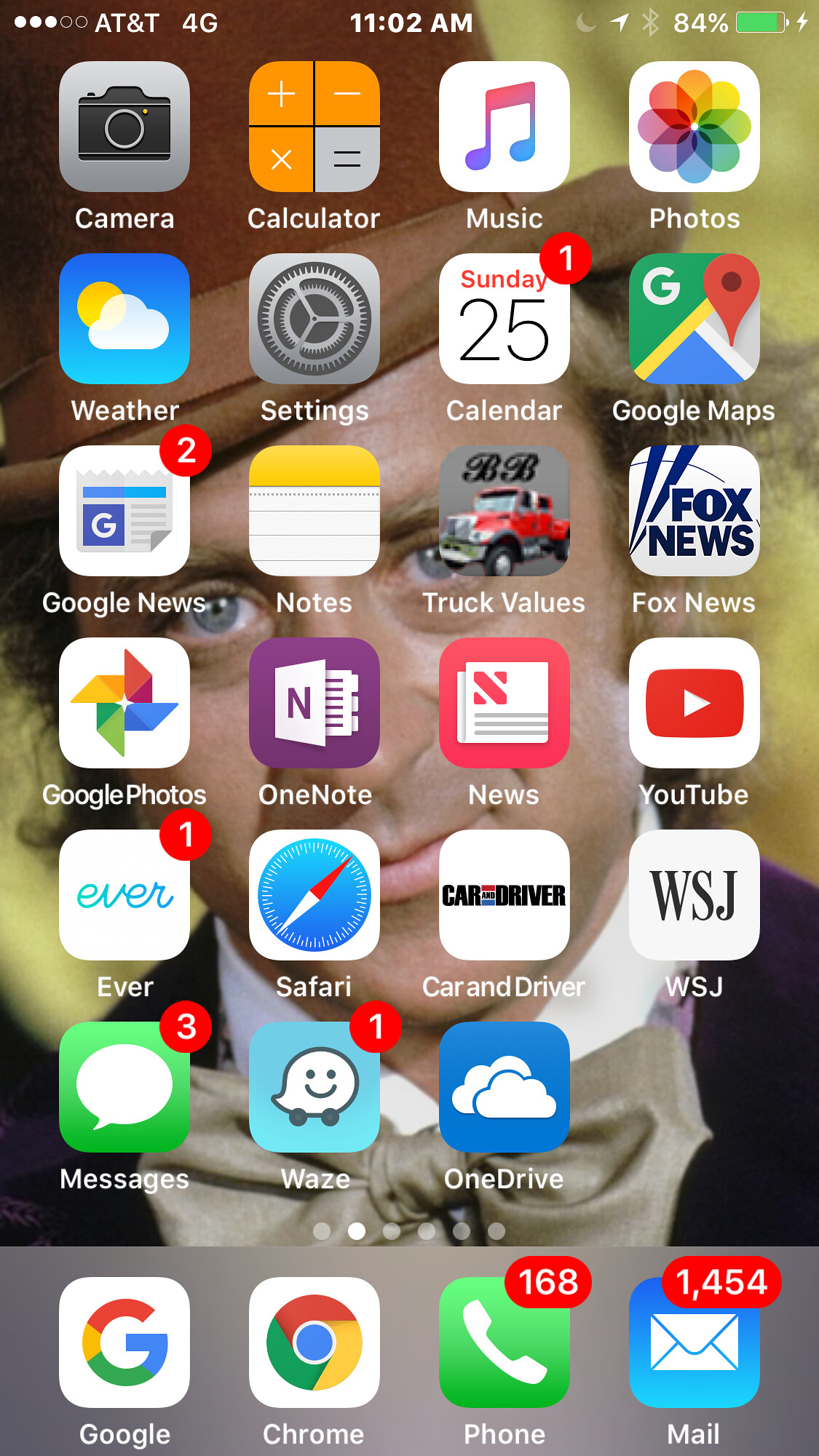This image captures the home screen of a smartphone, displaying a variety of apps organized across a single page. Notable apps include:

- Camera
- Calculator
- Music
- Photos
- Weather
- Settings
- Calendar (indicating Sunday the 25th)
- Google Maps
- Google News
- Notes
- Truck Values
- Fox News
- Google Photos
- OneNote
- News
- YouTube
- Ever
- Safari
- Car and Driver
- WSJ (Wall Street Journal)
- Messages
- Waze
- OneDrive

At the bottom of the screen, the dock contains:
- Google
- Chrome
- Phone
- Mail (with a red notification showing 1,454 unread messages)

The background features an image of a Caucasian actor.